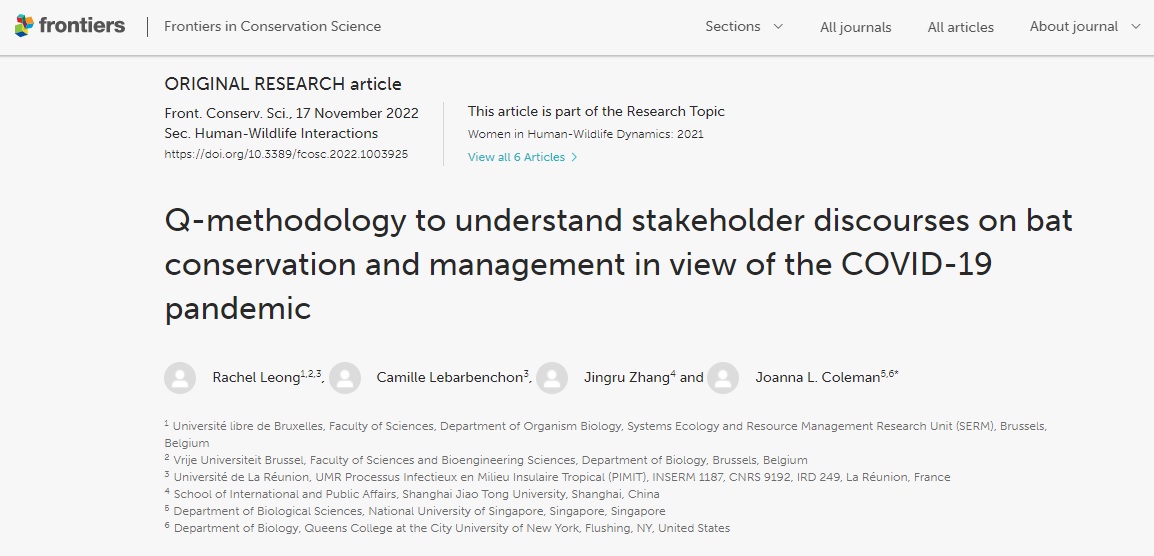This image depicts a webpage from the company "Frontiers," specifically from the "Frontiers in Conservation Science" journal, as indicated in the upper left-hand corner. The top section of the page features navigation tabs labeled "Sections," "Old Journals," "Old Articles," and "About Journal," all underlined by a gray line. The main content of the page is an original research article titled "Q methodology to understand stakeholder discourses on bat conservation and management in view of the COVID-19 pandemic," displayed prominently in large black letters.

Below the article title, several contributors are listed, each accompanied by generic profile icons. These names and their affiliations are listed in fine print, numbering from one to six, indicating their respective departments, primarily in the fields of biology and biological sciences.

The background of the website is a light gray color, providing a neutral backdrop to the text. Additionally, an icon located next to the "Frontiers" logo in the upper left-hand corner features a colorful design with elements in orange, blue, green, and yellow.